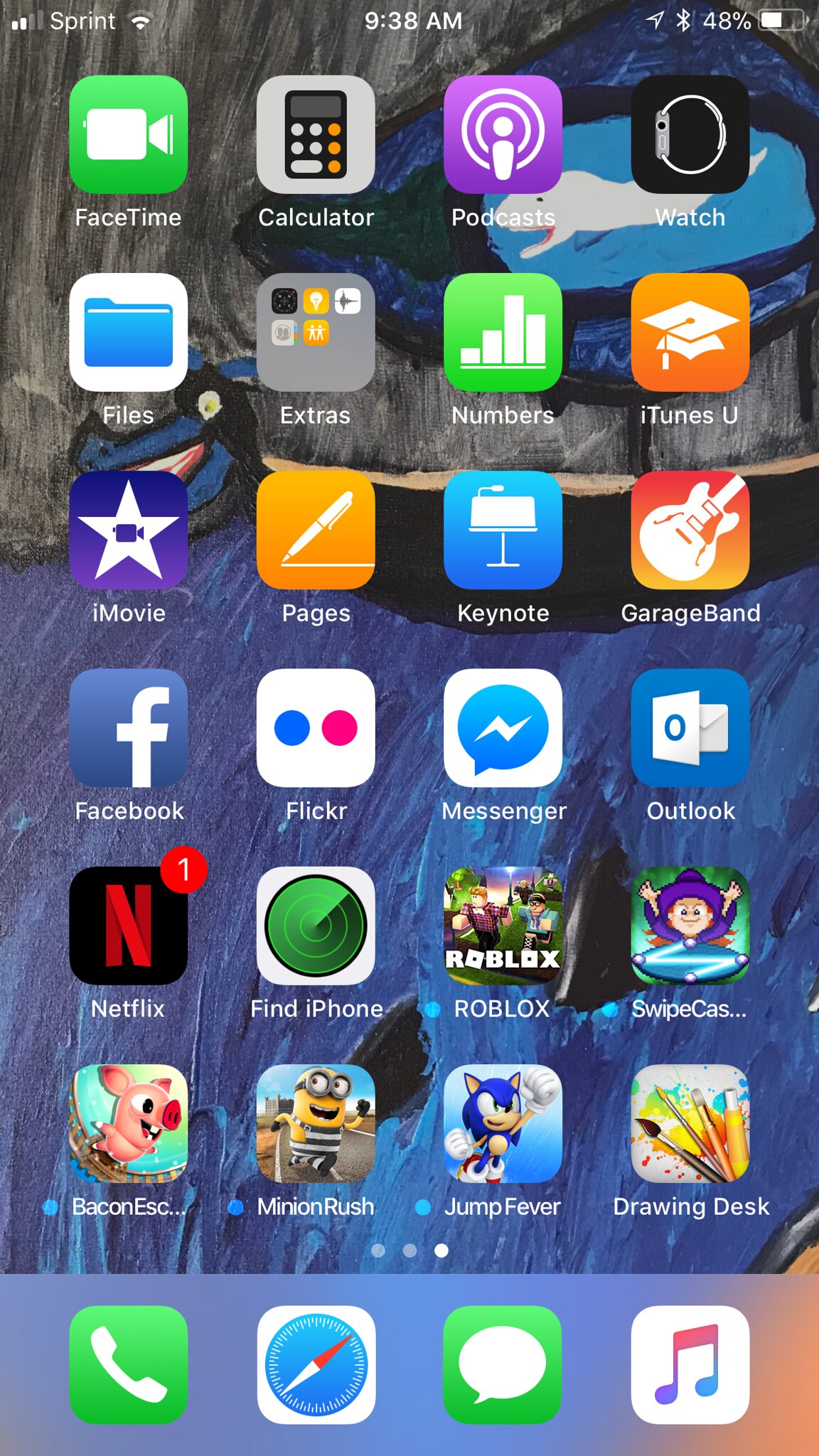This is an image displaying a screenshot of a cell phone's main screen. The top left corner of the screen shows a two out of four bar signal strength with "Sprint" indicated in white, followed by a two out of three bar Wi-Fi signal indicator. Centrally at the top, the time is displayed as 9:38 AM. The upper right corner contains a Bluetooth icon next to which is a battery icon showing 48% charge remaining.

The bottom of the image features a blue and orange-colored border containing four app icons: a phone icon, a compass icon, a text message bubble icon, and a musical note icon. The wallpaper on the screen illustrates a dynamic scene where a black boat with a dragon face at the front floats on blue water. The boat's sail, which features an image of a whale, rises into a gray sky.

The arranged apps on the screen, ordered from left to right, include:
- FaceTime
- Calculator
- Podcasts
- Watch
- Files
- Extras
- Numbers
- iTunes U
- iMovie
- Pages
- Keynote
- GarageBand
- Facebook
- Flickr
- Messenger
- Outlook
- Netflix
- Find iPhone
- Roblox
- Swipecast
- Bacon Escape
- Minion Rush
- Jump Fever
- Drawing Desk